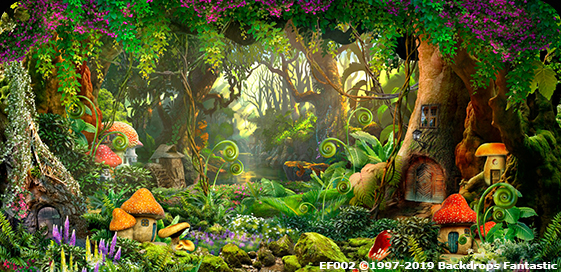This is a rectangular, cartoon-style digital image depicting an enchanting fairy forest. The vibrant scene is reminiscent of a whimsical gnome village or a magical Keebler elf town. Dominating the landscape are trees with built-in doors, one featuring an arched doorway, and small windows with four panes. Scattered throughout the forest are charming mushroom houses with colorful roofs—one with a distinctive red cap, another with a golden cap—each adorned with tiny green doors.

The forest is teeming with life and vivid colors not found in a typical woodland. Purple and yellow flowers are abundant, with lavender blooms adorning the hanging tree branches and the left foreground. Sun rays filter through the lush foliage, illuminating the greenery and casting a serene glow over a small stream or pond that runs through the center of the scene.

The overall composition hints at an idyllic, bustling community of mystical creatures. The bottom right corner of the image includes the text, "EF002, copyright 1997 to 2019, Backdrops Fantastic," indicating the creator of this fantastical artwork.